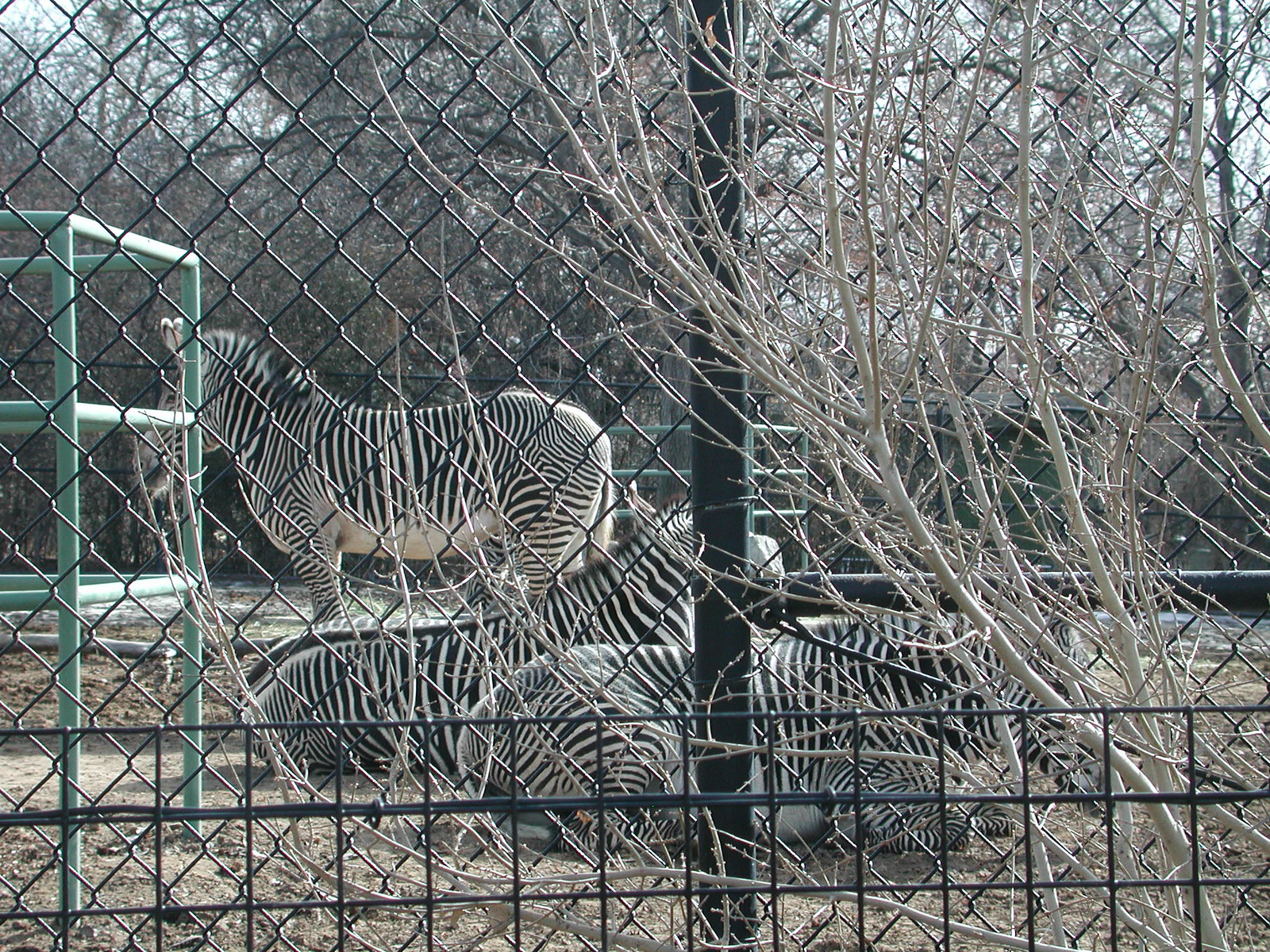In this detailed color photograph taken on an overcast day, three adult zebras—draped in their classic black and white stripes with pointy ears and a hint of fuzzy hair on their heads—are depicted within a zoo enclosure. Dominating the foreground are two zebras lying down on the bare dirt, both facing to the right. Behind them, a third zebra stands, gazing to the left. The zebras are enclosed by two types of fencing: a prominent black chain-link fence in the foreground, and a similar fence in the background separating them from a densely wooded area with bare grey branches. Positioned to the left within the enclosure is a green metal structure that resembles a playset or climbing frame. Dotting the foreground are clusters of saplings and spindly trees devoid of leaves, framing the scene in muted tones of beige, grey, and brown, with occasional patches of greeny-brown grass.